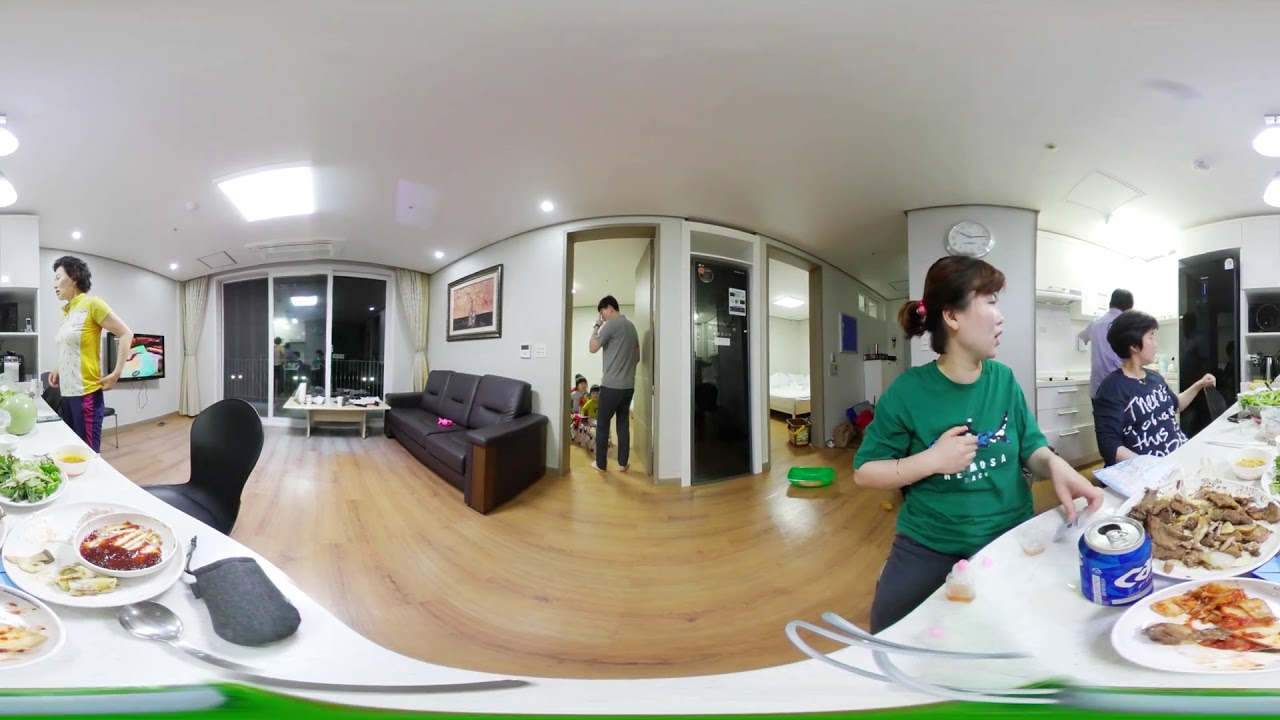In this vibrant and spacious setting, a family gathers for a grand dinner in what appears to be a well-furnished apartment or possibly a vacation beach house with a deck for relaxation. The scene is alive with the presence of variously dressed individuals in green, blue, yellow, gray, and lavender shirts, seemingly celebrating an occasion akin to a birthday party. The focal point is a long counter-like table draped with a white tablecloth, showcasing an eclectic spread of food, including dishes reminiscent of meatloaf, ravioli, wings, and Asian cuisine such as kimchi and beef, with drinks like Coca-Cola adding to the festive ambiance. The room features blonde hardwood floors and is filled with warm colors like green, white, gray, red, yellow, tan, pink, dark blue, light blue, and purple. The circular, panoramic view, enhanced by a fisheye lens effect, captures children playing with toys and a bike scattered around, while adults converse and relax. The large windows leading to a deck, the black sofa with a coffee table, and a painting on the wall add to the cozy, lived-in feel. In the background, a television is on, contributing to the casual and lively atmosphere of this indoor celebration in the late evening.